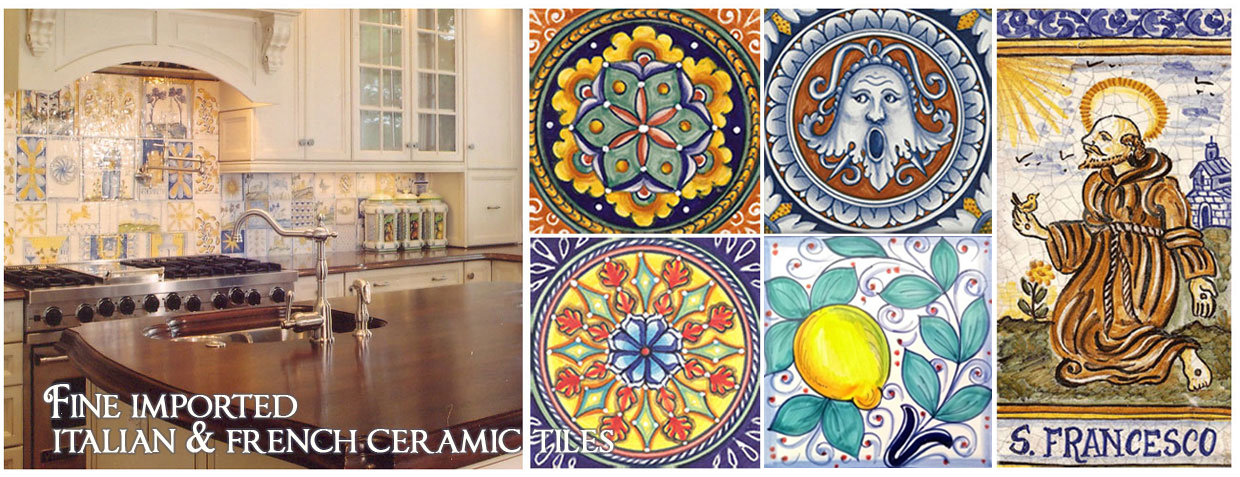The advertisement showcases fine imported Italian and French ceramic tiles. The primary image features a modern yet traditional farm-style kitchen with a central island, a stove with an overhang, and a wooden sink with a gold faucet. The backsplash behind the stove and countertop is adorned with a variety of intricate ceramic tiles. 

On the bottom right quadrant of the advertisement, a series of smaller images highlight individual tile designs. These include:
- A tile featuring a central leaf design that radiates outwards in red, green, blue, and yellow flower patterns, resembling an ornate crest.
- A tile with an orange background depicting what appears to be a ghost looking to the left, its mouth open as if in speech or song.
- A yellow-patterned tile in the bottom left quadrant with flower motifs that radiate outward.
- A tile depicting a vibrant lemon with green leaves.
- A tile labeled "San Francesco" showing a monk with a halo, a church in the background, a sun in the top left corner, and the monk dressed in a robe with a traditional rope belt, his head shaved.

These detailed depictions emphasize the artistry and variety of the fine ceramic tiles available for kitchen designs.